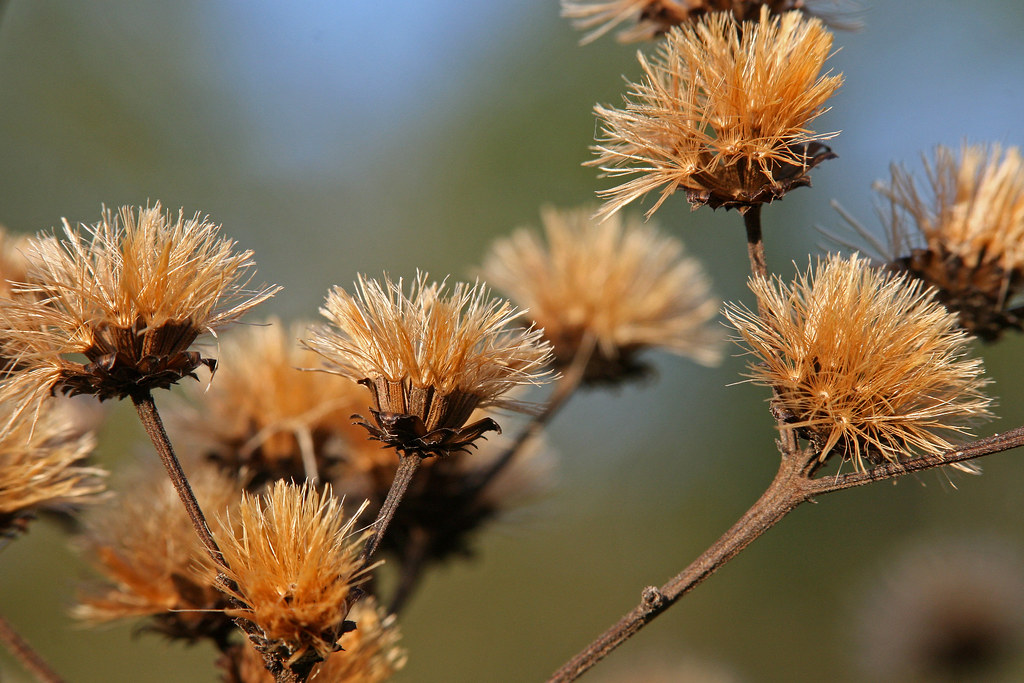This close-up photograph captures the intricate details of a dried-out, spiky plant, likely found in a desert region. The plant features multiple (specifically nine) thin brown stems emerging from a darker brown base. At the end of each stem are golden brown, spiky flower heads, resembling a tuft of spiked hair or even a party wig. The background is intentionally blurred, providing no additional context about the environment, although hints of blue suggest the presence of open sky and vague green blurs hint at distant vegetation. Despite the sunlit conditions, the plant appears completely dehydrated, with no moisture evident in any part of its structure.